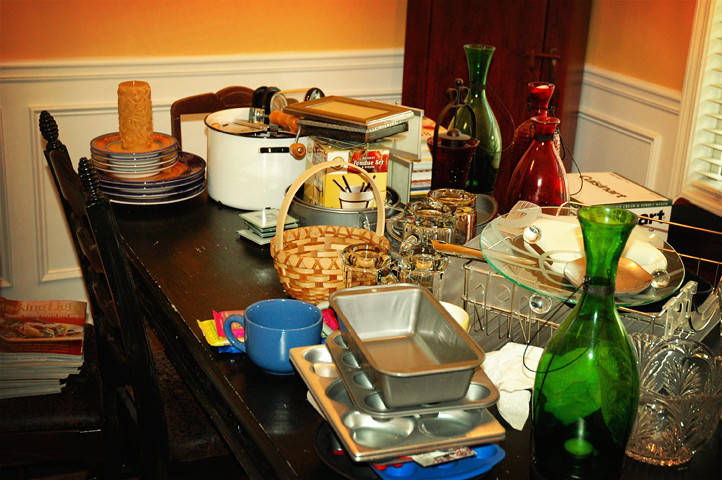In this vibrant color photograph, a cluttered dining room table is the focal point. The table is long and made of dark wood, paired with two contrasting chairs. One chair, matching the table's dark wood, features a backrest with two spires and a seat that appears to be cracked leather. The other chair, positioned on the opposite side, is shorter, crafted from a slightly lighter wood, and has a distinct design.

The dining room itself is framed by white wainscoting and golden yellow walls, creating a warm and inviting atmosphere. In the corner stands a tall, rectangular wood cabinet with a wooden latch. The room is illuminated by natural light filtering through the open white blinds.

The table's surface is a chaotic array of items. Stacked gold-colored plates vie for space with a blue coffee cup and several vases. Two of the vases are green, exuding an antique charm, while the other two are a striking red. Among the disarray, a black and white Cuisinart box and a crystal vase adorned with a leaf pattern stand out, adding to the eclectic mix of objects.